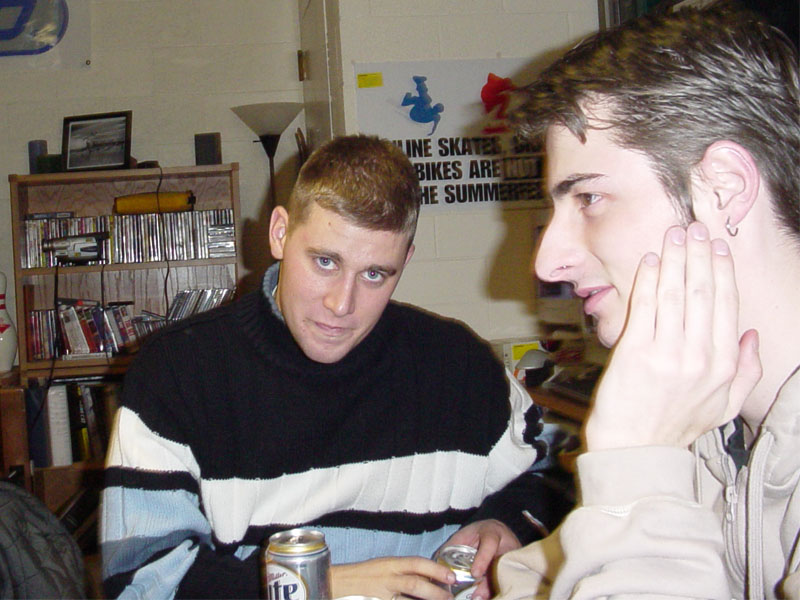The image depicts two young Caucasian men indoors, possibly in a college dorm room, as suggested by the brick-like wall in the background. On the left side of the image, there is a bookshelf cluttered with various items including books, DVDs, CDs, a camcorder, and a yellow bag, alongside a framed picture and a lamp. Centered prominently, one man with short blonde hair, light eyes, and a black, white, and blue striped sweater is holding a can of Miller Lite beer, gazing directly at the camera. To the right, another man with short dark hair, dark eyes, and an earring in his left ear, is wearing a beige hoodie and resting his chin on his left hand, looking off-camera. The candid, casual setting and their relaxed poses suggest an informal gathering or a moment of leisure.